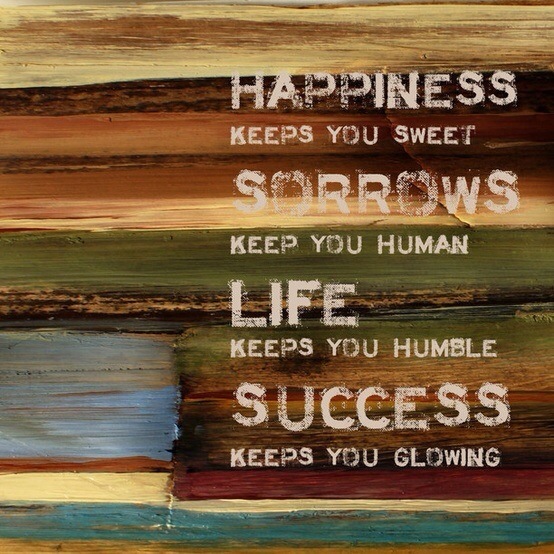The image showcases a horizontal wooden surface that has been intricately painted with various colors, revealing the natural brush strokes. The paint features layers of blue, white, brown, green, yellow, and different shades of dark and light browns. These colors are semi-transparent and lightly brushed, creating a visually rich and textured backdrop.

Along the right side of the image, white text appears in a mix of large and smaller fonts. The prominent words — "Happiness," "Sorrows," "Life," and "Success" — are in bold capital letters, with the phrases "keeps you sweet," "keep you human," "keeps you humble," and "keeps you glowing" displayed beneath them in a smaller, but similarly styled font. This sequence of words stretches vertically, making the message stand out against the colorful wooden background.